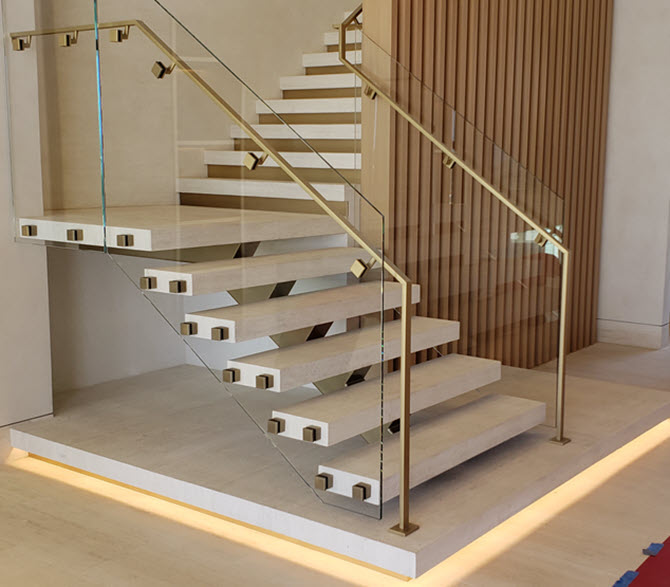This image captures a modern and meticulously clean indoor staircase. The staircase features white steps with brownish square knobs at the ends. It begins with five steps leading up to a landing, after which it ascends with more steps in a left-right configuration. The stairs themselves are somewhat distinct and separated from each other. The banister is made of brass or gold with clear glass or acrylic sides, giving it a sleek, contemporary look. The flooring beneath the staircase appears to be white but has been described differently as tan or gray with decorative elements. The raised platform beneath the first few steps is particularly eye-catching, described as gray or silver, and seems to have a subtle illumination or orangish-yellowish lighting effect. Moreover, the image captures a brown wall made of vertical slats of wood to the right of the staircase, adding texture and a warm contrast. Vertical brown blinds can also be seen on this wall. Overall, the staircase is set in a square frame, highlighting its elegant design and sophisticated aesthetic.